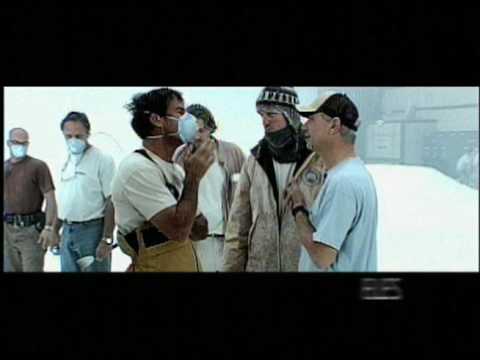The photo, set in a horizontal rectangular frame with black horizontal bars at the top and bottom, captures an outdoor scene dominated by a crowd of middle-aged men, predominantly white, in casual attire, with short-sleeved shirts and pants. Most are wearing face masks—blue disposable ones—typically used during the COVID pandemic. Prominently in the foreground, an unmasked white man wearing a baseball cap, blue t-shirt, and a watch on his left wrist, converses with a mask-wearing man of darker skin tone dressed in a white t-shirt and khaki pants. Additionally, another man in the crowd, wearing a jacket, scarf, and beanie, suggests colder weather, augmented by possible snow and overexposed white hotspots in parts of the background. There is also a partially visible building in the upper right corner. Another man with his right arm raised stands at the center, adding to the dynamic interaction within this scene of social engagement.